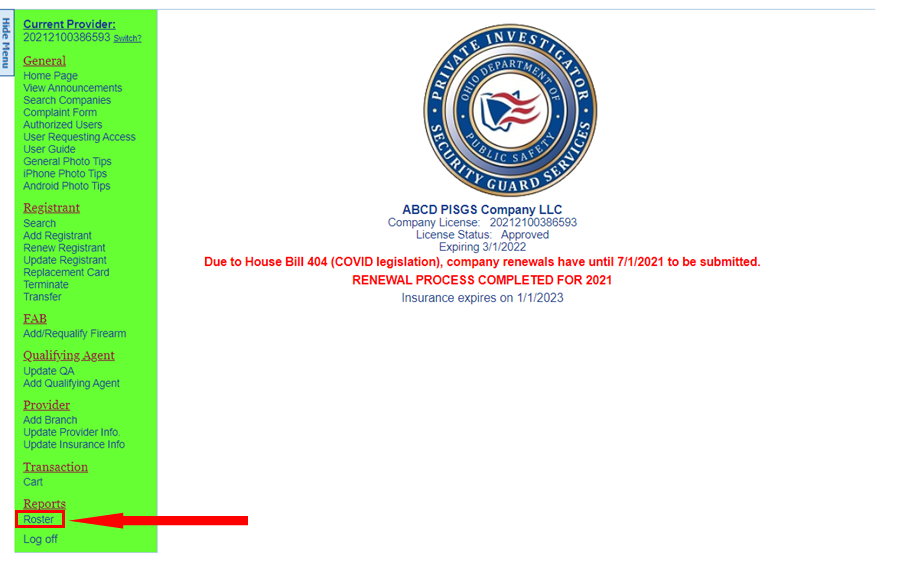The image depicts the official seal of the Ohio Department of Public Safety's Private Investigator Security Guard Services (PISGS). The seal is circular with multiple concentric circles and is primarily blue and gold with a touch of red in the center. At the core of the seal lies an outlined representation of the United States flag.

Encircling the central emblem, the first ring is blue with the text "Ohio Department of Public Safety" printed in white. The next layer forms a whitish-bluish band, followed by a narrow blue ring on the perimeter, which bears the text "Private Investigator Security Guard Services" in white lettering.

Beneath the seal, the text reads:
"ABCD PISGS Company LLC
Company License: (License Number)
License Status: Approved
Expiring: 3-1-2022"

In red ink is a notice:
"Due to House Bill 404 COVID legislation, company renewals have until 7-1-2021 to be submitted. Renewal process completed for 2021. Insurance expires on 1-1-2023."

On the left side of the image is a green bar featuring several links, including:
- Current Provider
- General (Home, View Announcements, Search Companies, Public Photos, etc.)
- Registrant (Search/Add Registrant, Renew Registrant, etc.)
- FAB (Add/Re-qualify Firearm, Qualifying Agent, Provider Transaction, Reports)

Under "Reports," a prominent red arrow points toward a section labeled "Roster," which is also outlined in red. The image seems to provide detailed information and links pertinent to security and investigative services.